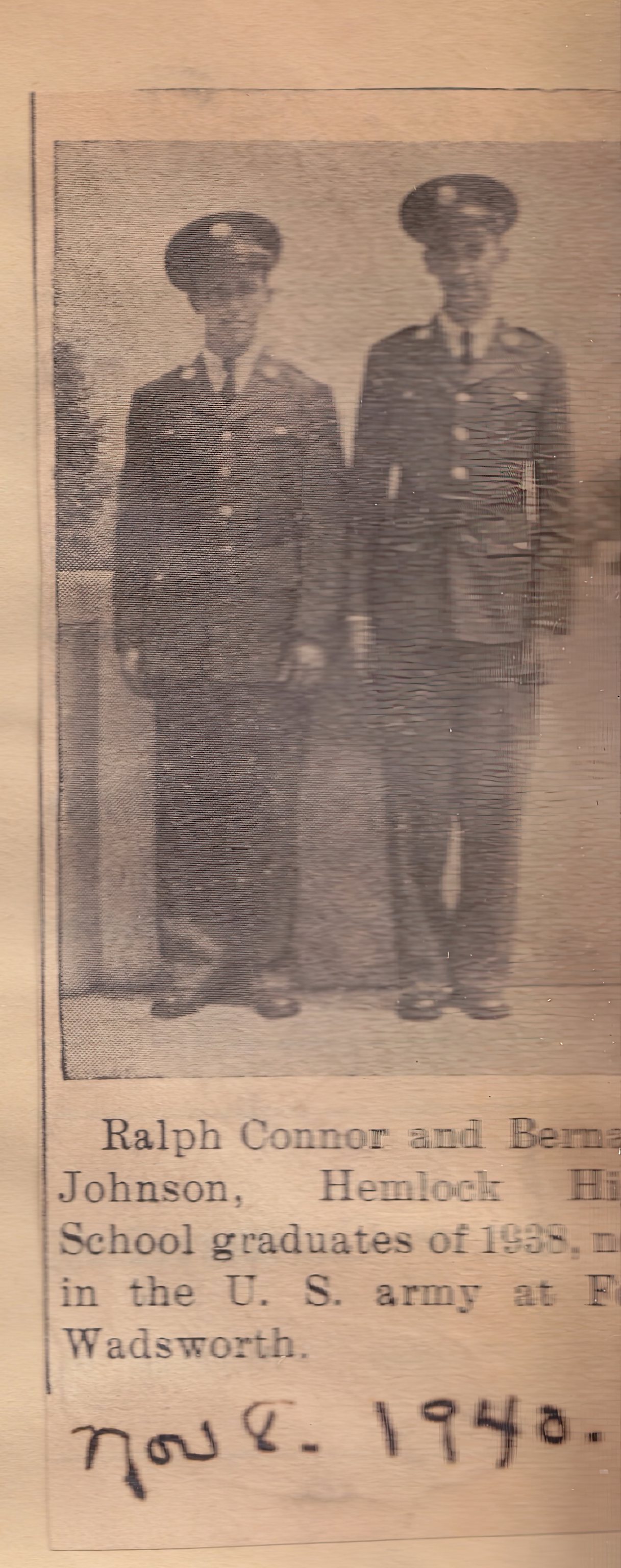This portrait-oriented image appears to be a weathered and faded newspaper clipping, featuring a cream or light tan background indicative of its age. The top 60% of the snippet displays a black-and-white photograph of two young men dressed in military uniforms, complete with hats, coats, and visible suit ties. The men stand straight against a plain backdrop, one noticeably taller than the other. Below the photograph, black text provides partial identifications, reading: "Ralph Conner and Bernie / Johnson Hemlock," followed by "school graduates of 1938" and continues with "in the US Army at Wadsworth." The date "November 8, 1940" is written by hand in ink, annotating the clipping. This snippet likely announces the military service of these two 1938 graduates.